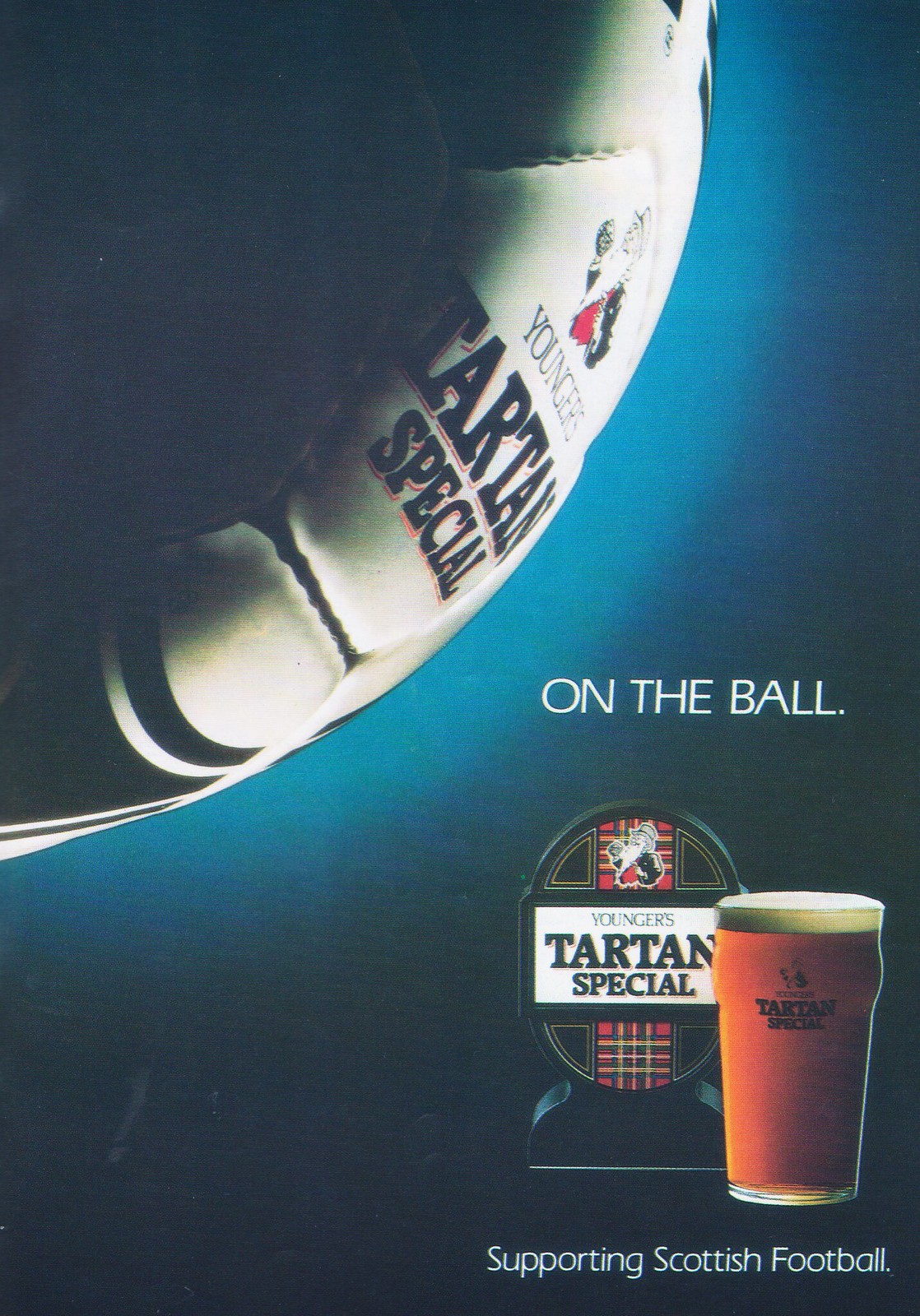The image is a rectangular advertisement for Younger's Tartan Special beer. Dominated by a blue background with gradient shades that deepen to a nearly blackish blue at the bottom, the ad prominently features a large soccer ball on the left side. The ball's right side is illuminated, displaying the text "Tartan Special" in black font, while the rest remains in shadow. To the right of the ball, bold white text in all caps reads "ON THE BALL." Below this, there is a detailed depiction of a glass filled with golden beer, adorned with the Younger's Tartan Special logo alongside a bust of a man with a beard and top hat. At the bottom right corner, the message "SUPPORTING SCOTTISH FOOTBALL" is clearly displayed in white text.